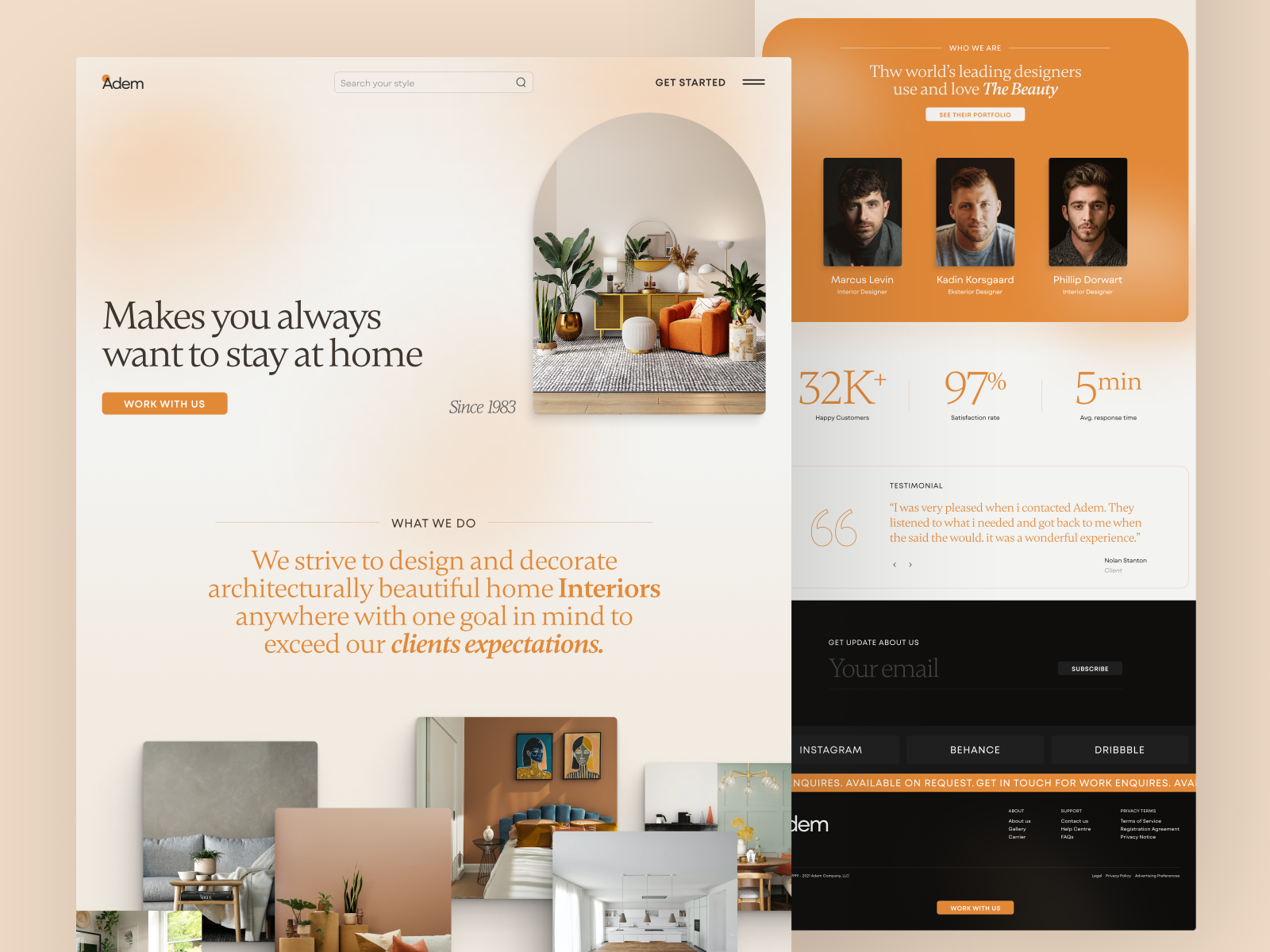This image is a screenshot from a website in a split background format. The left side and the far right edge of the background are beige, while the section past the center towards the right has a white background. At the top, there is a yellow-orange pop-up with a headline that is intended to say "The world's leading designers love the beauty," but it contains a typo and reads "thw world's leading designers use in love."

Below this pop-up, there is a feature section titled "Third Portfolio" showcasing three designers: Marcus, an Interior Designer; Caden Korsgaard, an Exterior Designer; and Philip Dorwan, another Interior Designer. 

Underneath this, on a gray background, there are key statistics about the service: "32k+ happy customers," a "97% satisfaction rate," and a "five-minute average response time." This is followed by a testimonial area.

A black banner towards the bottom prompts users to "Get updates about us" with fields for entering an email to subscribe. Social media icons for Instagram, Behance, and Dribble are also included.

An orange banner further down invites users to engage: "Inquiries available on a quest to get in touch for work inquiries."

On the left side of the screenshot, there is an image of a living room with a caption saying "Makes you always want to stay home." Below this, there is a section titled "What We Do" accompanied by more images from different clients.